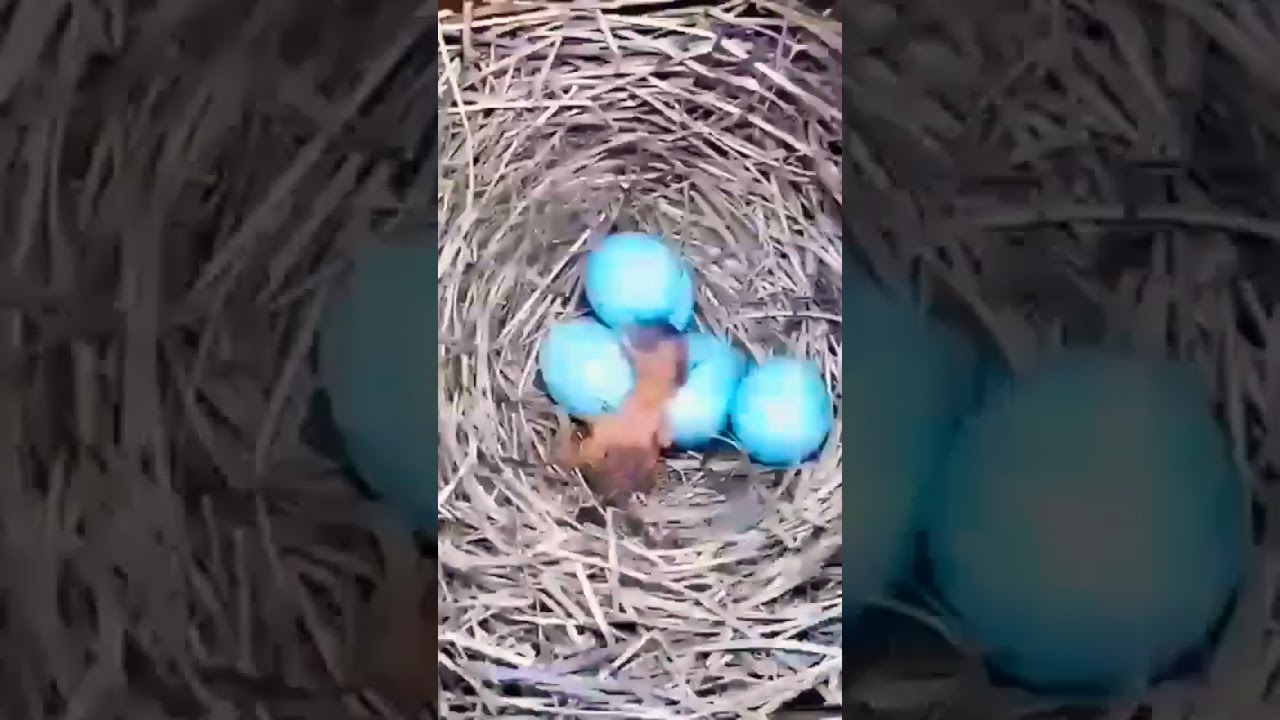This is a photograph of a robin's nest, capturing a close-up view of its intricate construction made from dried plant materials, leaves, and twigs. The nest cradles four bright, sky-blue eggs arranged with three in a row and one positioned nearby. Nestled among the eggs is a newly hatched chick, its tiny pink body and small wings visible as it faces away from the camera, with its head nestled between the eggs. The image appears slightly blurry, almost as if it's a screenshot from a video. The vertical photo features a prominent close-up of the nest centered in the middle, with a darker, expanded version of the image as the background.